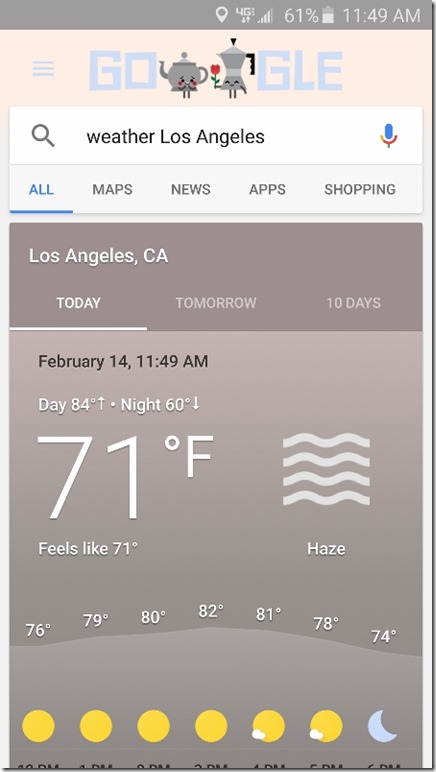The image captures a screenshot of a Google search conducted on a smartphone. At the top of the screen, the Google logo is creatively illustrated with the second "O" replaced by a pair of teapots, each adorned with faces, one of which holds a flower. Below the whimsical logo is the search query "weather Los Angeles," typed in the search bar.

Beneath the search bar, the interface displays various categories such as "All" (highlighted and underlined in blue), "Maps," "News," "Apps," and "Shopping." The user has selected "All," leading to a detailed weather report for "Los Angeles, CA."

The weather report is segmented with options for "Today," "Tomorrow," and "10 days," with "Today" currently selected. The date is specified as February 14th, and the time shown is 11:49 a.m. The detailed forecast reveals a daytime high of 84°F and a nighttime low of 60°F, while the current temperature is listed as 71°F, feeling like 71°F with hazy conditions. At the bottom of the screen, there are icons depicting phases of the moon and associated temperature details.